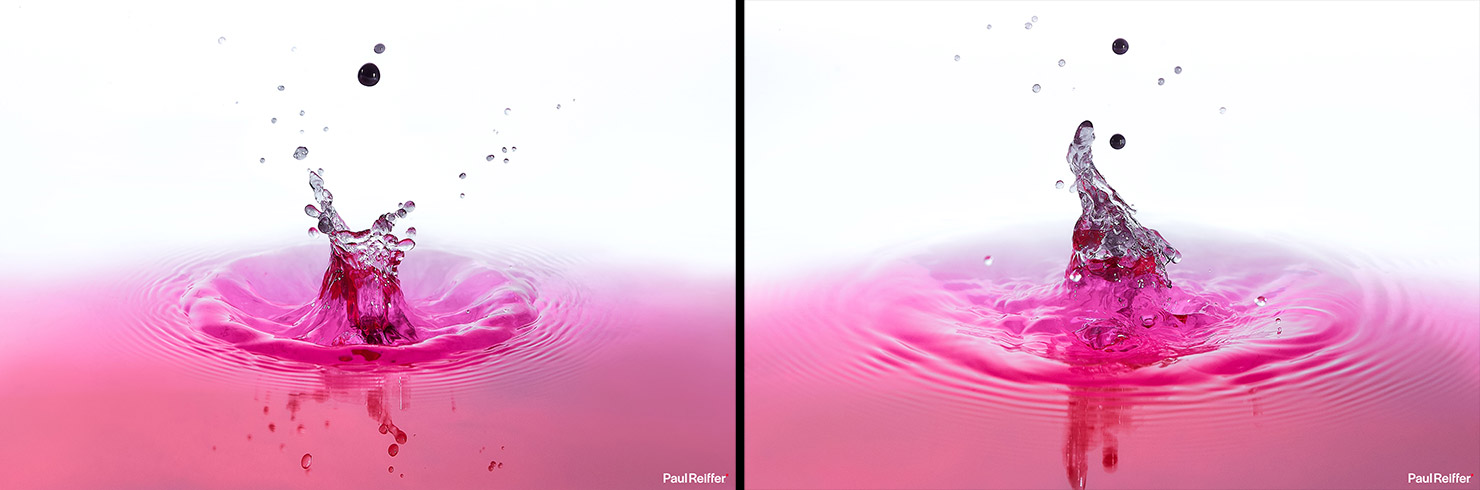The image showcases a pair of strikingly similar yet distinct pictures, both depicting a vibrant scene of pinkish-purple water. In the left image, the water forms a circular shape with prominent ridges, and various bubbles and droplets can be seen splashing upwards. The right image mirrors this composition but with a subtle difference: the water droplets at the top have coalesced into a shape reminiscent of a horn, further accentuated by additional droplets. Both images emanate a sense of dynamic motion and fluid beauty. The artist or photographer's name, likely Paul Raffner or Ruffner, is subtly inscribed in the bottom right corner, attributing the captivating work to its creator.